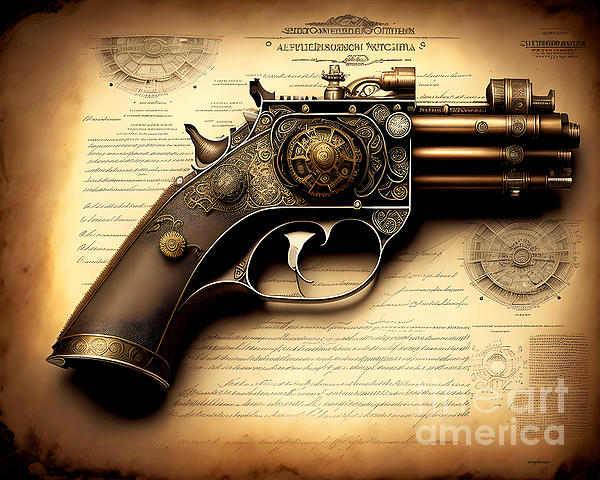The image features a highly ornamented, antique-style revolver with a distinct steampunk aesthetic. The side view showcases the gun's intricate design, which includes engravings in gold, silver, copper, and brass. The revolver, depicted in bronze hues, boasts baroque features and an elaborate, wheel-like mechanism near the trigger. 

Behind the revolver is an aged, brownish parchment with black cursive text and diagrams, likely in a foreign language. The parchment adds to the old-world feel, featuring seals in the corners and creating an orange and yellow gradient across the paper. 

In the bottom right corner of the image, there's a watermark that reads "Fine Art America" in white text. While the image appears hyper-realistic, it is actually a computer-generated depiction, blending elements of antique weaponry with futuristic design elements.